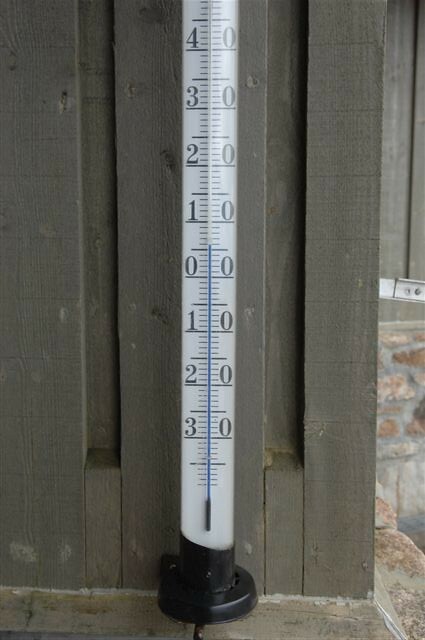This photograph captures a close-up view of a vertically mounted thermometer. The thermometer features a slender, white strip affixed to a circular, black base that rests on a gray-painted, wooden surface. The backdrop of the image displays vertically oriented wood paneling in a muted gray shade. At the bottom of the frame, a stone ledge is visible, supporting the black base of the thermometer and extending to the right edge, where it meets a small section of a stone wall. Above this intersecting stone wall, the continuation of the gray-painted wooden surface is visible.

The thermometer itself is marked with horizontal black lines and numerals. On its left side, the scale is labeled from top to bottom with the numbers 4, 3, 2, 1, 0, 1, 2, 3. The right side of the thermometer shows repeated zeros, appearing eight times. A thin, blue indicator line on the thermometer rises to a point just above the 0 mark on the left scale, aligning approximately halfway between 0 and 1. This detailed composition highlights the precise measurements and the context of the surrounding environment, providing an intricate look at the placement and functionality of the thermometer.